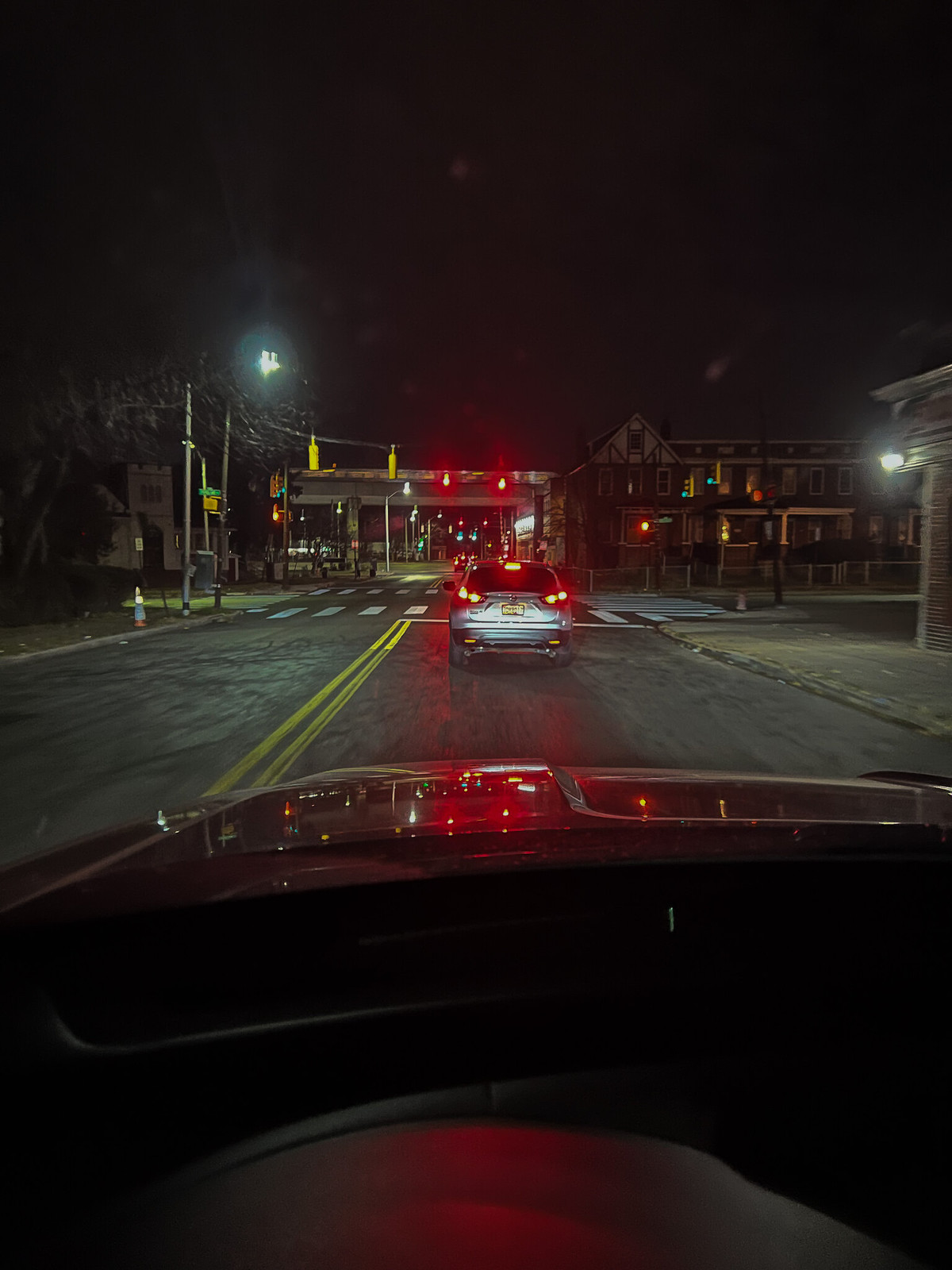The image captures a nighttime scene from a driver's perspective, looking out onto a traffic-filled street. The dashboard, a blend of gray and black, is visible at the bottom of the frame, leading up to the windshield. The road ahead is gray, featuring two solid yellow lines that divide the opposing lanes of traffic. Directly in front of the vehicle is a white crosswalk, followed by a grey SUV with its red taillights illuminated. Above the SUV, a set of traffic lights glows red.

On the right side of the image, there is a dark brown building. To the left of this building, a gray bridge extends into the distance, and further left, another house is visible. The night sky is pitch black, playing a stark contrast against the street and the illuminated elements. Finally, a streetlamp stands on the right side of the frame, casting light onto the scene below.